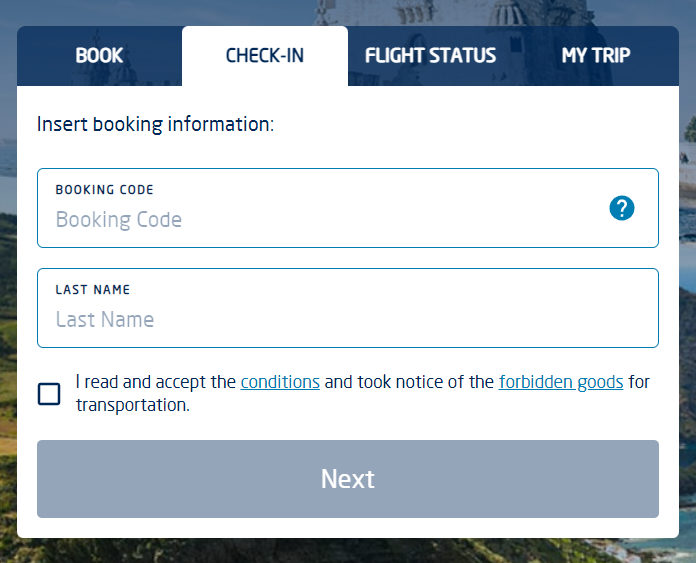The image depicts a user interface on a travel website, where the background features a vibrant mix of landscapes, including farmer's fields, grassy areas, and potentially a seascape, all melding into a picturesque sky. Overlaid on this scenic background is a dominant user interface section focused on travel booking and check-in functionalities.

At the top of the interface are four clickable tabs:

1. **BOOK** (blue background, white uppercase letters)
2. **CHECK-IN** (white background, black uppercase letters, highlighted as it's currently selected)
3. **FLIGHT STATUS** (blue, semi-transparent background, white uppercase letters)
4. **MY TRIP** (blue semi-transparent background, white uppercase letters)

Beneath the currently selected **CHECK-IN** tab, there is a prominent white box section. On the left side, black text instructs users to "Insert booking information."

Within this section:

- A thin blue-rimmed box labeled "BOOKING CODE" appears at the top left in blue uppercase letters. Beneath it, finer blue text repeats "Booking code," and to the far right is a blue circle with a white question mark icon.
- Below this, another faint blue-rimmed box is labeled "LAST NAME" (upper left, blue uppercase letters). Inside, finer letters repeat "Last name."
- Adjacent to these fields is an unchecked blue square checkbox. Beside the checkbox, black and blue text reads, "I read and accept the conditions" (with "conditions" underlined and hyperlinked), followed by, "and take took notice of the forbidden goods for transportation" (with "forbidden" and "goods" also underlined and hyperlinked).

At the bottom of this interface section is a large, faint blue button with "NEXT" written in white letters. This button is currently grayed out, indicating it is not yet clickable.

The detailed layout and the specific clickable elements are designed to facilitate the travel booking and check-in process efficiently.